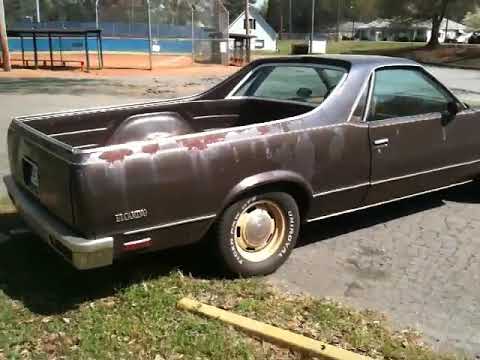This outdoor image captures a very old, rusting brown Chevrolet El Camino with a weathered, faded paint job. The vehicle, identifiable by the "El Camino" emblem on its lower-right side, exhibits notable rust particularly on its back end. Though only the rear and part of the side profile are visible, it's clear this El Camino, characterized by its unique combination of a car front and truck rear, has seen better days. The truck is parked on a pavement near a grassy area bordered by a yellow curb. In the background, to the left, there's a pool area enclosed by a fence, with the blue of the pool and a small white building visible. To the right and further in the background, another grassy expanse features a tree, with adjacent white houses nestled among more trees, all suggesting the setting is a park. The overall image is blurry, adding to its nostalgic atmosphere, reinforcing the aged appearance of both the car and the scene.